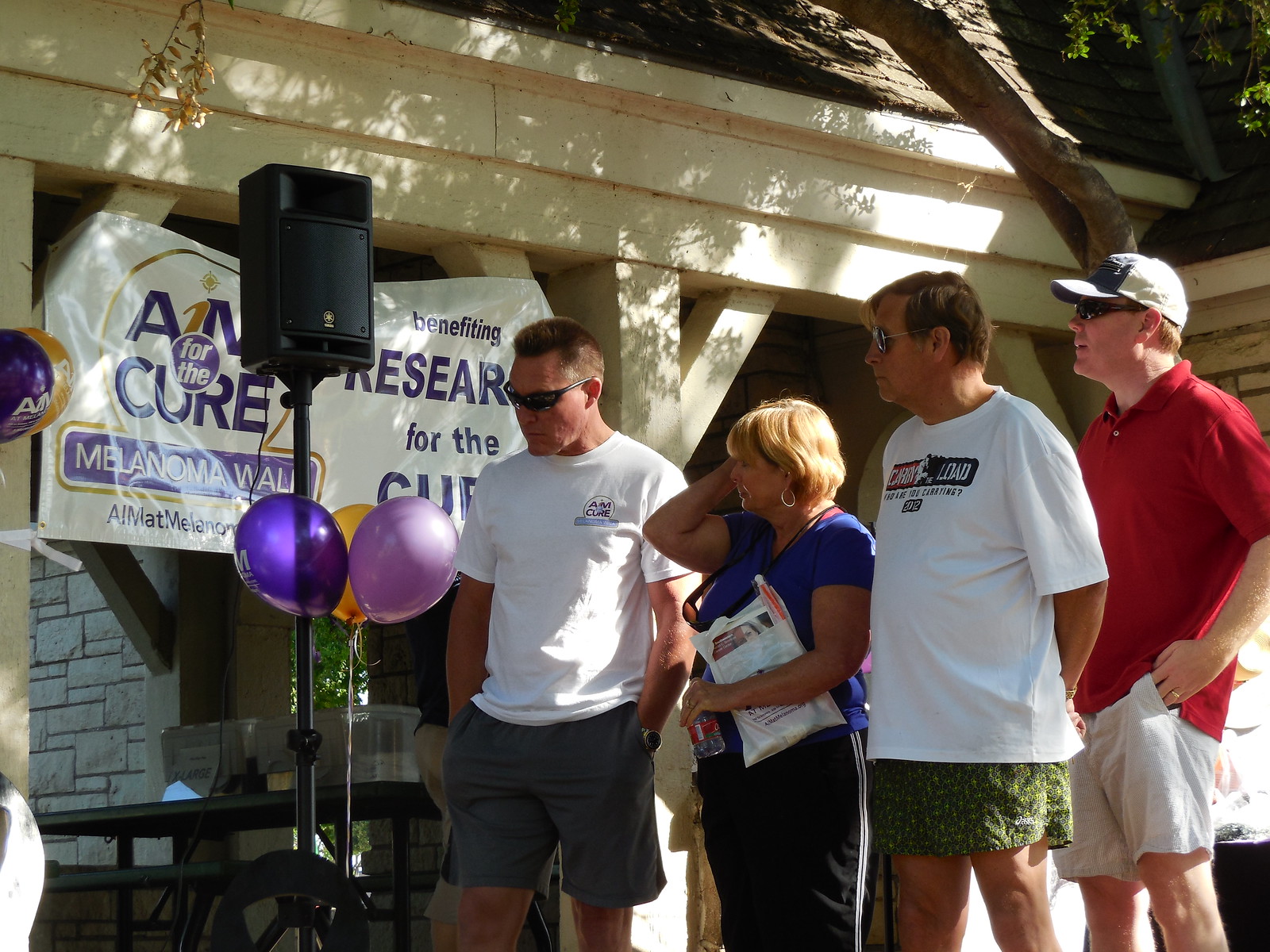In this outdoor image, a small group comprising three men and one woman stands informally in front of a building adorned with a white-and-purple banner. The banner reads, "Aim for the Cure, Benefiting Research for the Cure, Melanoma Walk," indicating a fundraising event, likely for melanoma research. The people are casually dressed in T-shirts and shorts or track pants, with one man notably wearing a red short-sleeved shirt and khaki shorts. In the foreground, a black speaker mounted on a pole is decorated with festive balloons in shades of bright purple, lavender, and gold. The group's attention is directed to the left side of the image, though the focus of their gaze is not visible. The setting is well-lit by natural daylight, and the building behind them features a mix of stone cladding and wooden porch elements, enhancing the casual and welcoming ambiance of the event.